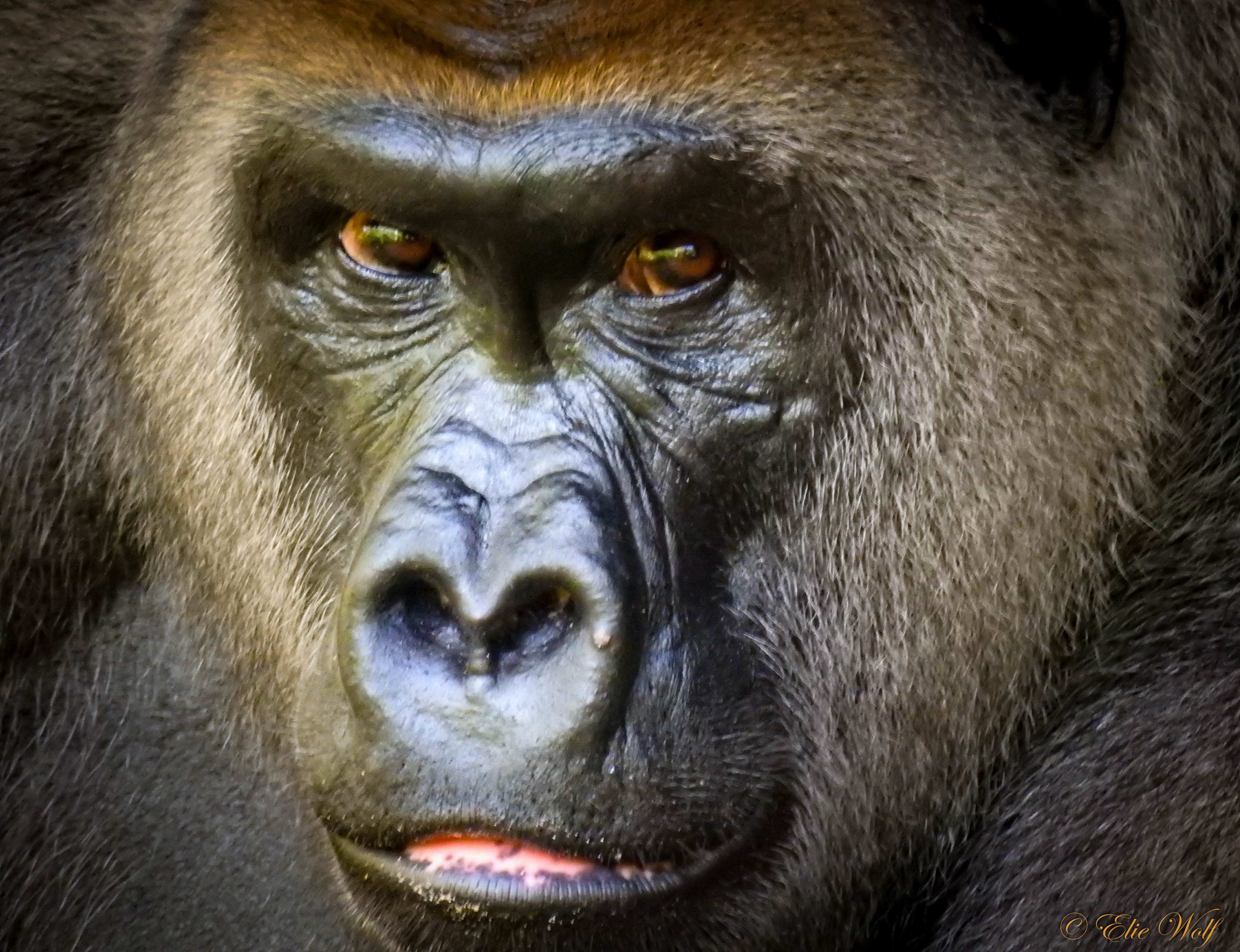This image features an extremely close-up shot of a gorilla's face, likely a male given its prominent facial features. The gorilla's fur forms a heart-shaped frame around its face, transitioning from a dark black to a lighter brown and blonde around the edges. Its leathery, nearly fur-free face has a strikingly smooth, black texture. The gorilla’s deep brown eyes, framed by a slightly lighter brow ridge, gaze intently just to the right of the camera. Slightly open, its mouth reveals pink lips with a hint of dirt. Minimal fur is present around the facial area, with a touch of gray in the beard. Sunlight highlights the gorilla's nose, suggesting the photo was taken during the daytime. In the bottom right corner, the photographer’s name, "Ellie Wolfe," is inscribed in thin, gold cursive, marking the image's copyright. The overall impression is one of somber intensity, as the gorilla gives a serious, contemplative look toward the viewer.